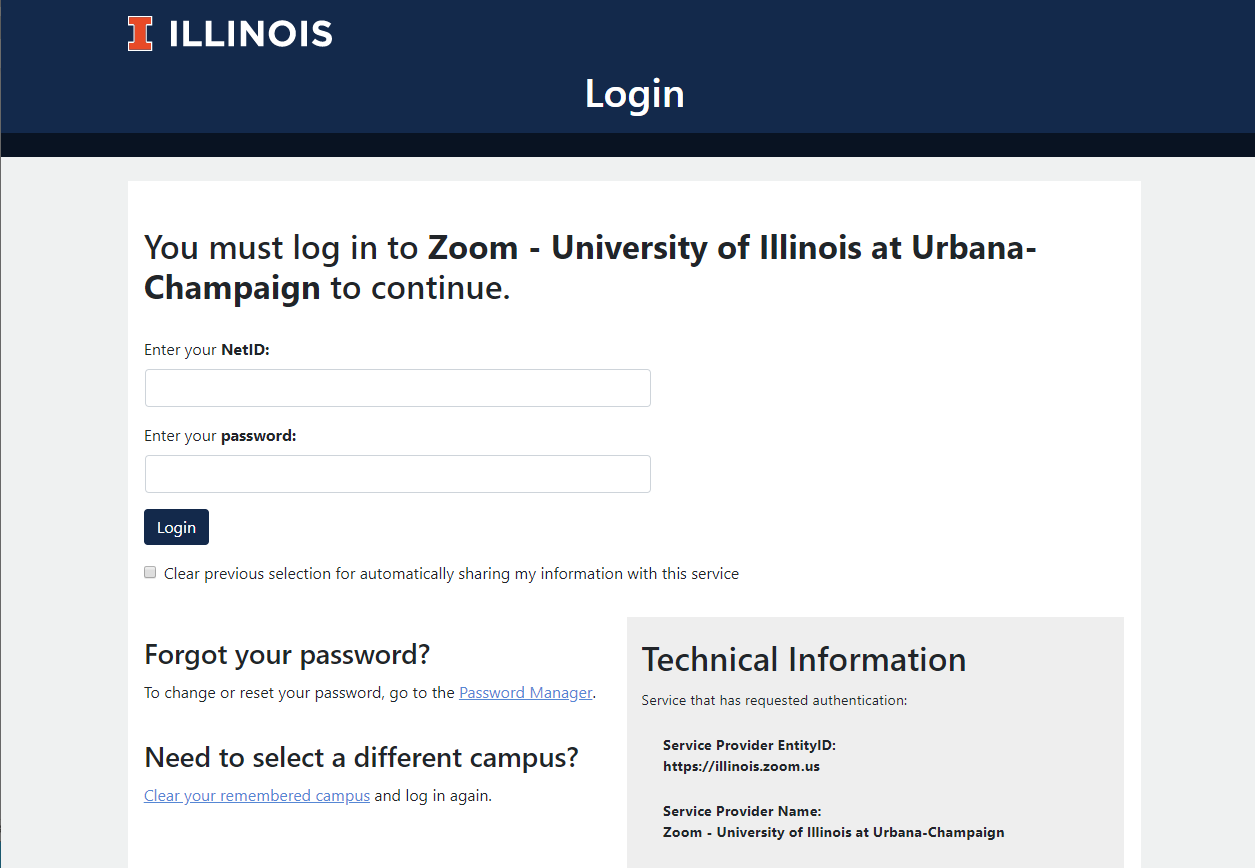A cropped screenshot of a web page features a login section from the University of Illinois at Urbana-Champaign's Zoom portal. The website employs a blue, grey, and white color scheme. The dark blue header at the top prominently displays a red-bolded letter "I" logo adjacent to the word "Illinois" in white text. Centered in the header is a "Login" title in white text.

Below the header, there is a grey section containing a white form box. The form is titled, "You must log in to Zoom University of Illinois at Urbana-Champaign to continue." It includes two input fields for the user's net ID and password. A dark blue "Login" button is situated below these fields. Additionally, the section provides hyperlinks for users who have forgotten their password or need to select a different campus. The overall design is clean and straightforward, focusing attention on the login functionality.